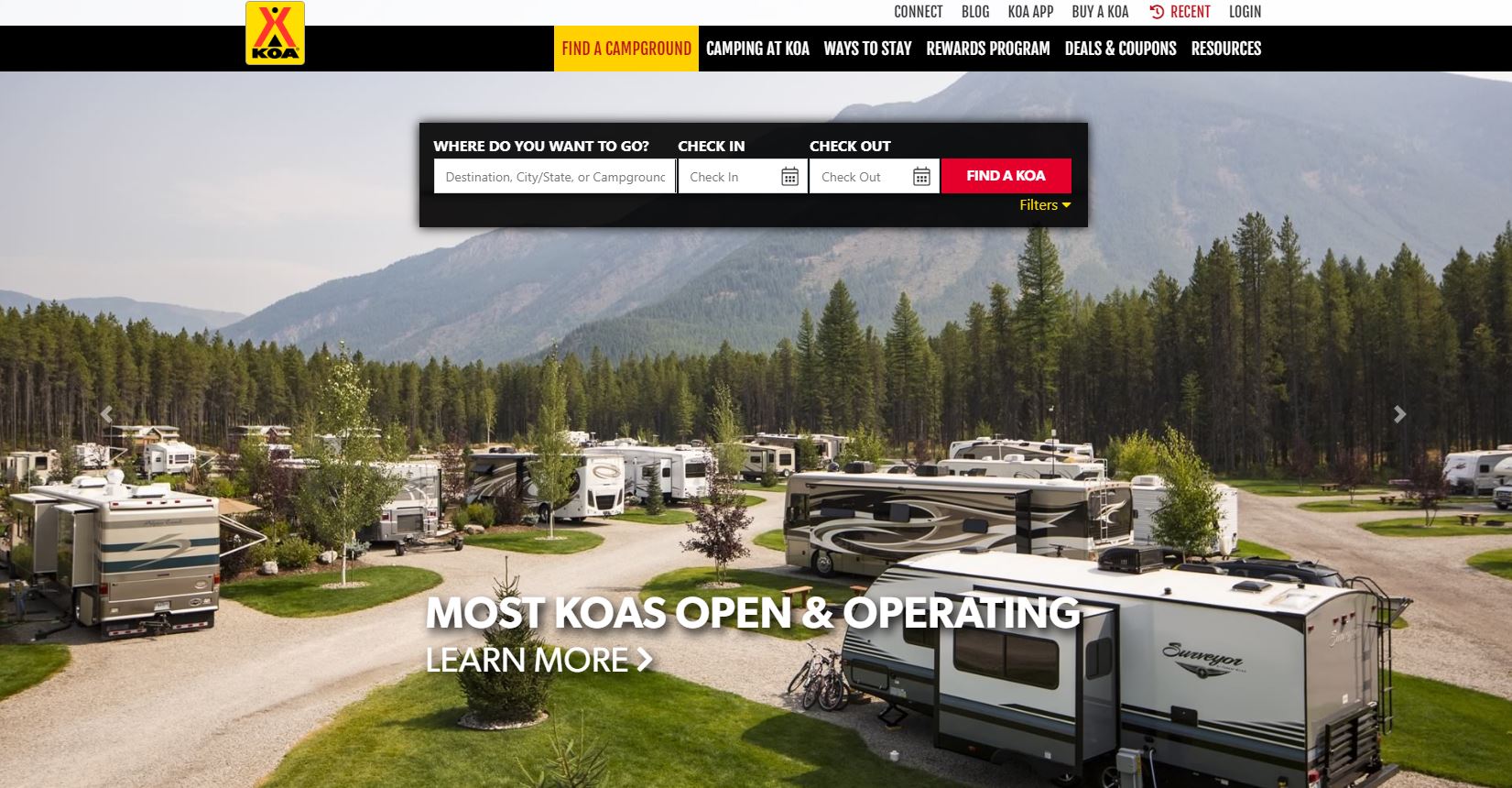**Detailed Caption**:

The image is a screenshot of the website for KOA (Kampgrounds of America) camping grounds, captured in landscape orientation. It appears to be taken on a laptop. Starting from the upper left and stretching slightly to the right is a white stripe labeled "Connect Blog." Adjacent to this, towards the center-right, the website header reads "happy-camping.koa.app" in black, with "Recent" highlighted in red, followed by a "Log In" option. 

Below this, a black stripe runs horizontally, featuring the KOA logo on a yellow background towards the left—a stylized tent icon. Adjacent to the logo are various navigation tabs including "Find a Campground," "Camping at KOA," "Ways to Stay," "Rewards Program," "Deals and Coupons," and "Resources." The "Find a Campground" tab is highlighted in red, indicating the current selection.

The next section showcases an expansive background image occupying the entire screen. The upper left-hand corner of this image features a gray, overcast sky, perhaps intended to be sunnier but presenting a more subdued atmosphere. The backdrop includes a rugged mountain range, descending to a lush, verdant forest of green pine trees occupying the midsection.

Dominating the center and bottom of the image is a panoramic view of a mobile home park, where campers can park their RVs. At the top section of this park scene is a black input box asking, "Where do you want to go?" Users can enter a destination, city, state, or specific campground here. Below the input box are check-in and check-out calendars, followed by a red "Find a KOA" button. Additional filters for searches are located beneath this button. A footer note states, "Most KOA locations are open and operating," with a prompt to "Learn More," situated at the very bottom of the image. 

This descriptive caption aims to provide a thorough overview of the webpage components, ensuring the visual layout and navigation elements are explicitly detailed.